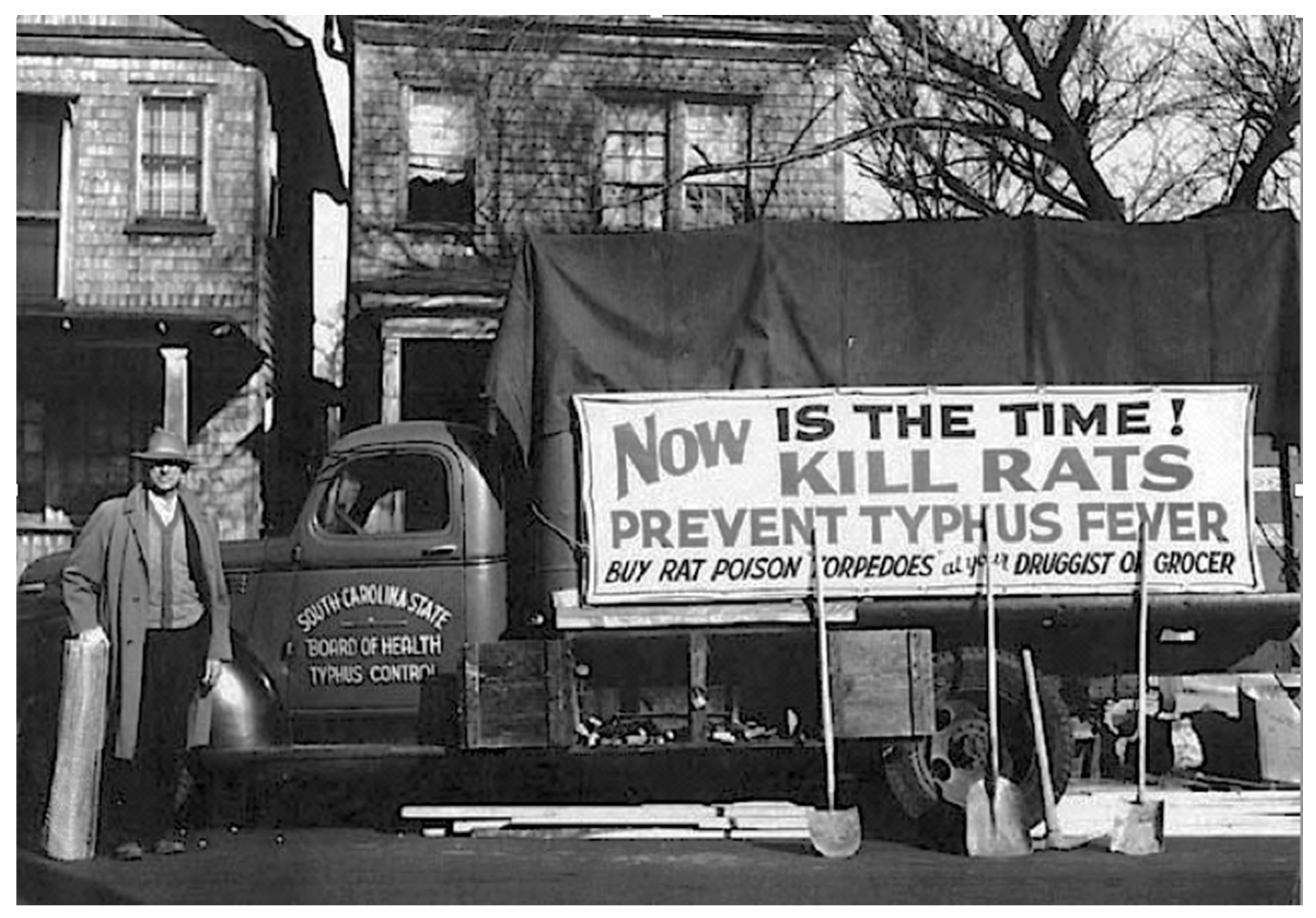The black and white photograph captures a historical scene in front of what appears to be a residential building with old wood paneling. A man, dressed in an overcoat, hat, and sweater, stands with his hands in his pockets, looking directly at the camera. He is positioned beside an old-style commercial truck with a wooden crate bed. Printed on the door of the truck is "South Carolina State Board of Health, Typhus County." The bed of the truck prominently features a large sign that reads, "Now is the Time to Kill Rats, Prevent Typhus Fever, Buy Rat Poison Torpedoes at your Druggist or Grocer." Leaning against the truck are multiple shovels, indicating tools for yard or garden use. In the background, two houses and a stark, leafless tree add to the vintage atmosphere of the scene.